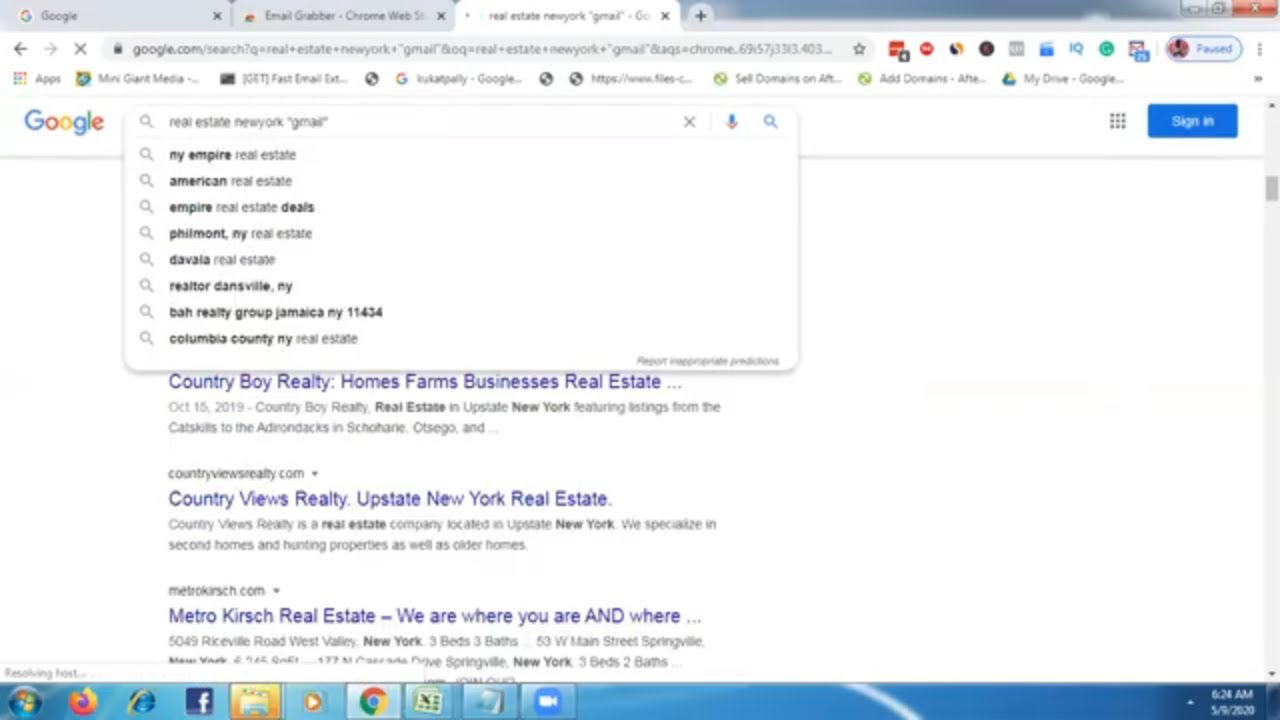A detailed descriptive caption for the image:

"This is a screenshot of a person's computer monitor displaying a Google search for 'Real Estate, New York, Gmail.' The search bar is populated with various suggested search queries including 'New York Empire Real Estate,' 'American Real Estate,' 'Empire Real Estate Deals,' 'Philmont New York Real Estate,' 'Davala Real Estate,' 'Realtor Dansville New York,' 'Baa Reality Group Jamaica NY 11434,' and 'Columbia County New York Real Estate.' 

Below the search bar, snippets of various real estate ads and listings are visible. One such listing mentions 'Country Boy Realty' with the tagline 'Homes, Farms, Businesses, Real Estate' and an accompanying date 'October 15, 2019.' The ad further describes 'Country Boy Realty' as specializing in real estate in Upstate New York, featuring listings from the Catskills to the Adirondacks including areas like Schoharie and Otsego, with the text continuing with an ellipsis indicating more content.

Another listing for 'Country Views Realty' advertises real estate services in Upstate New York, saying it specializes in second homes, hunting properties, and older homes. The ad includes a website address, 'CountryViewsRealty.com,' and a brief description about the company.

A further snippet mentions 'Metro Kirsch Real Estate,' with the partial tagline 'We are where you are and where...' and an incomplete address '5049 Brightsville Road, West Valley, New York, Three Beds, Three Baths, 53 West Main Street Springville,' with additional text cut off at the bottom.

The monitor's taskbar is visible at the bottom of the screenshot, displaying the time as '6:24 AM' alongside the date as '59, 2020,' suggesting an evident error or partial cut-off in displaying the correct date."